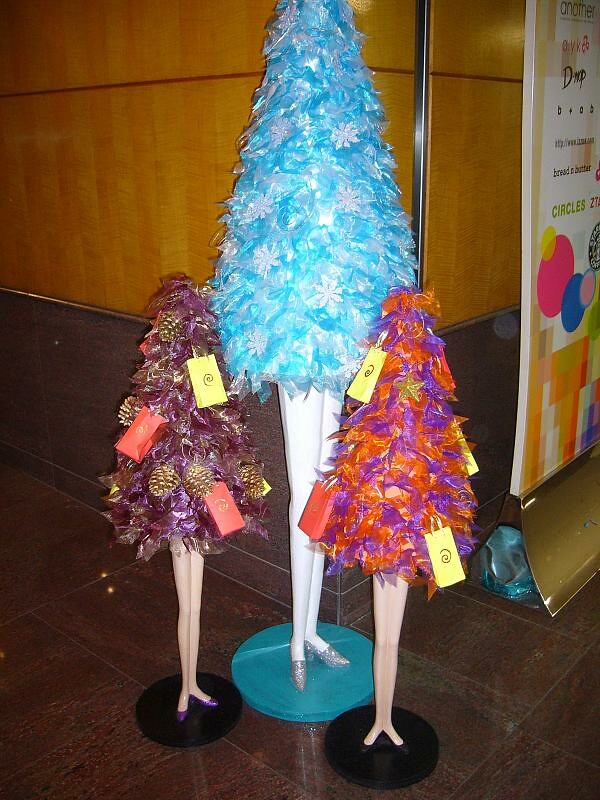The image features an indoor display of three mannequins dressed as Christmas trees, positioned against a detailed wooden wall. The lower portion of the wall is dark brown, possibly granite, while the upper portion is a polished lighter brown with a red line running horizontally across it. The floor is dark brown tile, matching the wall's lower half. To the right, there is a square banner featuring red, blue, and light pink circles, resembling ice cream cones, with text that includes a website and the words "another B+" and "bread and butter."

In the foreground, two smaller mannequins stand on black circular platforms. The mannequin on the left is adorned as a purple Christmas tree, decorated with red and yellow small bags, and brown pine cones, standing on white legs with purple shoes. The mannequin on the right is a more vibrant orange and purple tree, also featuring red and yellow mini shopping bags, on white legs with black shoes. The larger mannequin in the back stands on a teal circular platform, dressed as a light blue tree with white snowflake designs, grey sparkly shoes, and white mannequin legs.